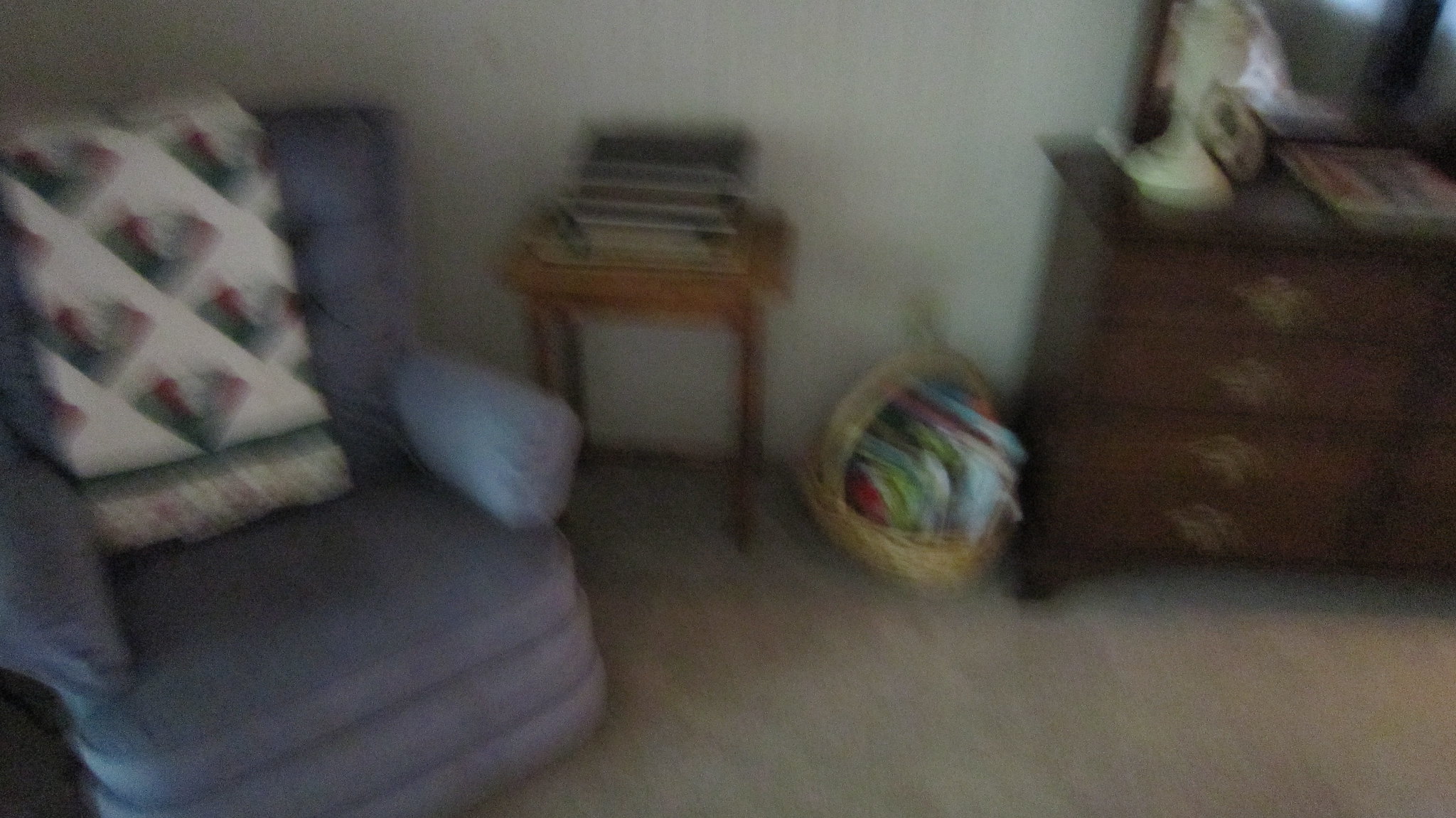This image captures a nostalgic living room scene, albeit in a blurry and unfocused manner. The room features a beige carpet and centers around a vintage, single-seater love chair reminiscent of 1980s furniture. The chair is baby blue with tufted cushions that are buttoned, creating a poofy, textured appearance, and a folded quilt drapes over the backrest. Adjacent to the chair is a wooden TV dinner tray, stacked with several books. A light, woven basket, similar to those used for Easter, sits next to the tray and appears to contain children's items like books or wooden puzzles. To the side, there is an older-style dresser, more commonly found in bedrooms. It has gold-toned emblems on the drawers and a ceramic head sculpture placed on top, adding a touch of character to the living room decor.